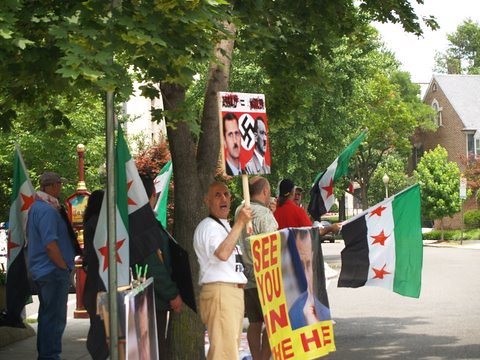In this image, the scene is set during a daytime protest along an asphalt street lined with trees, conveying an outdoor setting. The focal point is a group of people, positioned centrally, holding various signs that express hateful messages. Notably, several protesters are waving Syrian flags, with at least six or seven flags visible. One man stands prominently in the foreground, dressed in a white t-shirt and khaki pants, holding a picket sign. His sign features an image of President Bashar al-Assad with a small Hitler mustache on the left, juxtaposed with Adolf Hitler on the right, set against the backdrop of a Nazi flag with a swastika. To the top left of the image, residential homes and additional greenery are visible, while the colors throughout the scene include gray, green, white, red, black, yellow, and blue. This image captures the intensity and atmosphere of a politically charged protest.